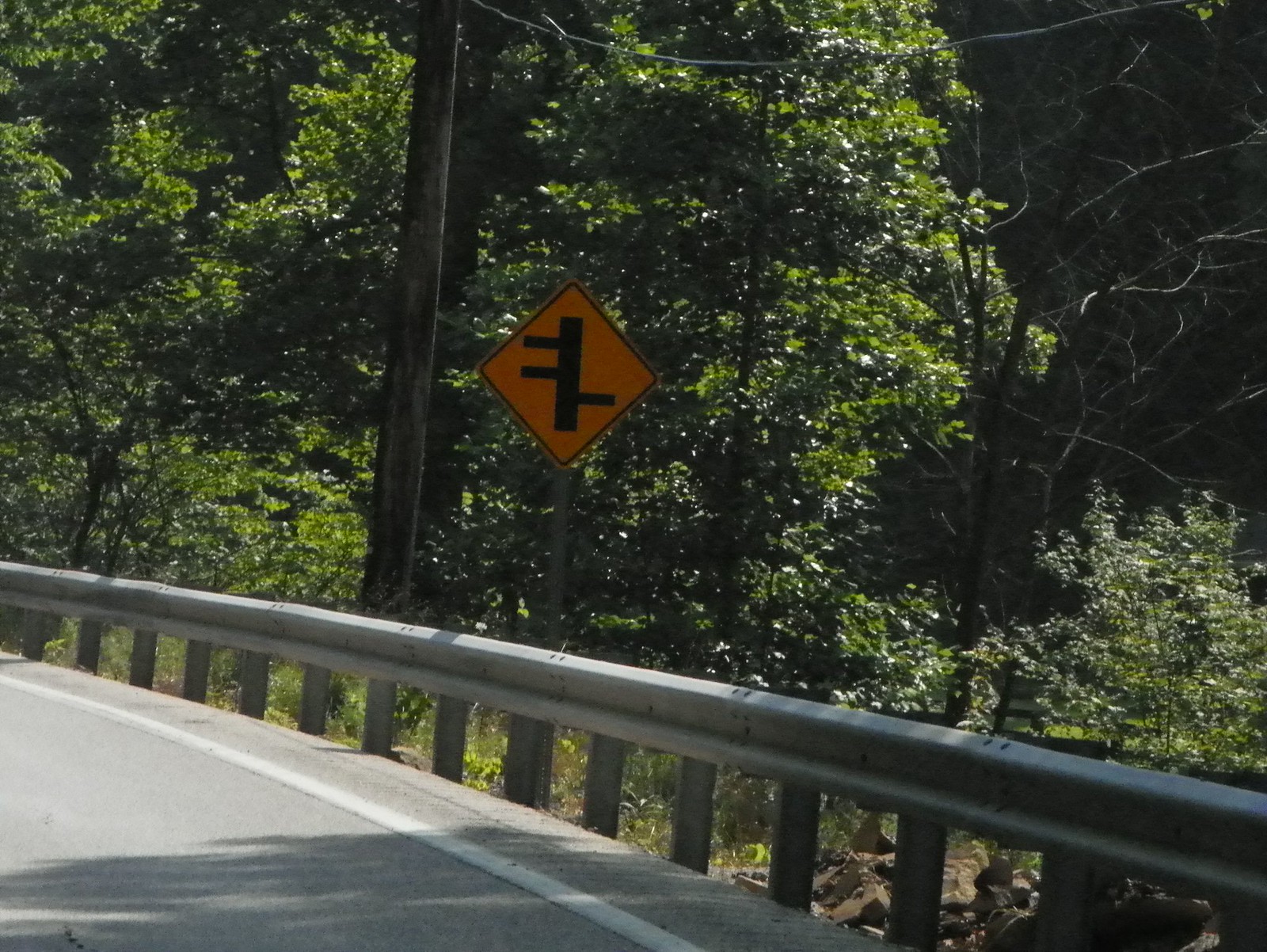A winding grayish road, featuring a white stripe along its side, extends through the landscape. Adjacent to the road is a series of small, gray posts topped with a metallic grayish-silver rail that runs the entire length of the image. Beyond the rail, dense green trees form a natural boundary. Among the trees, a large brown utility pole stands out, with a drooping cable attached to it. A distinctive yellow diamond-shaped sign with a black line intersecting vertically and additional lines diverging to the left at the top and to the right at the bottom is prominently displayed. On the right side of the image, a few leafless, dead trees contrast against the greenery. A shadow cast by a tree to the right stretches across the road, adding depth to the scene.